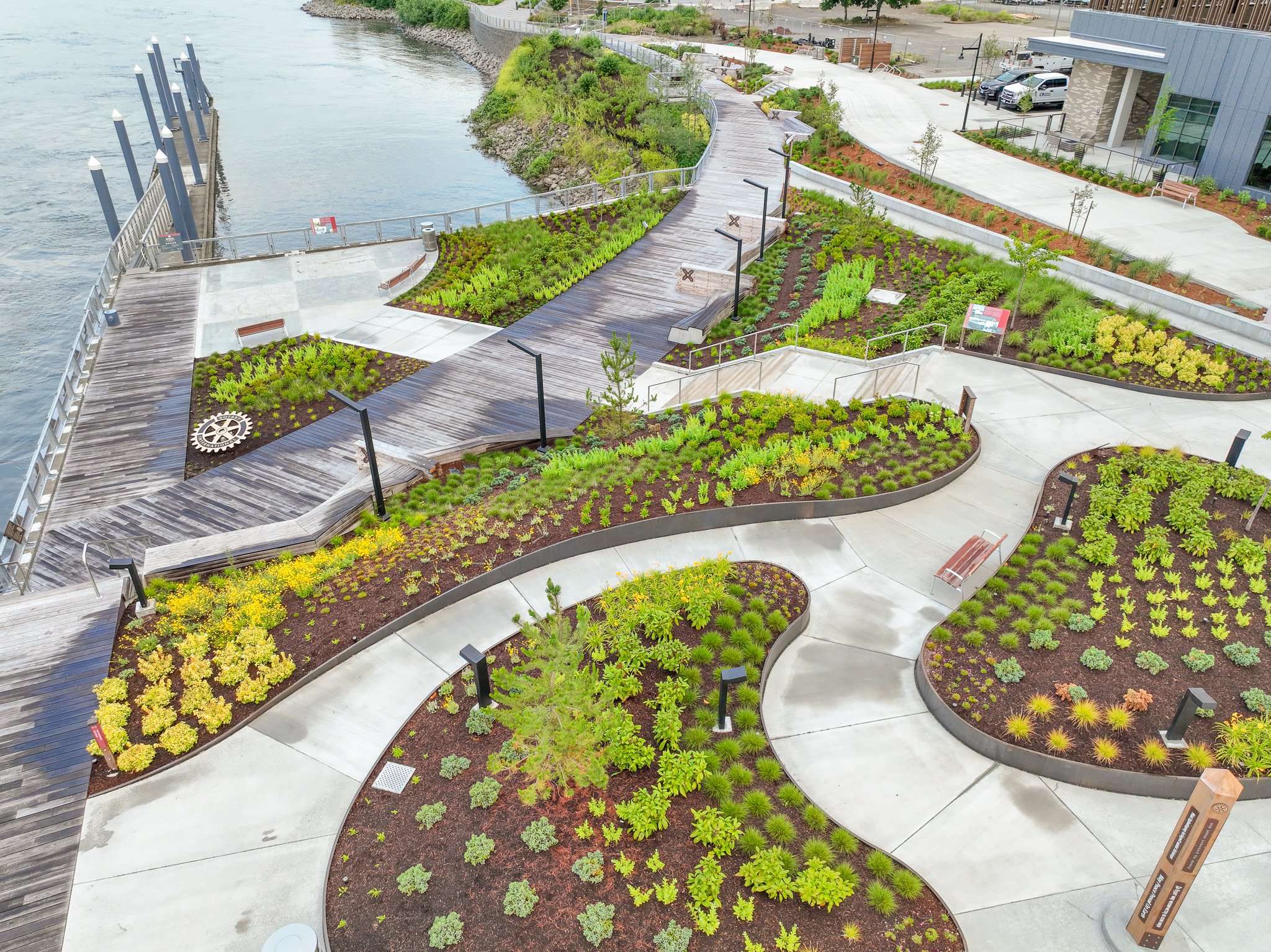An aerial view captures a meticulously planned garden adjacent to a scenic boardwalk along a tranquil body of water, possibly a bay or lake. The boardwalk is constructed with gray boards and features an intriguing diagonal section that continues parallel to the waterfront. At the heart of the image are six asymmetrically shaped gardens, each resembling elongated ovals with smoothly rounded edges. These gardens are artistically arranged in tiers, showcasing a diverse array of flora.

The planting design is strikingly structured: lines of vibrant flowers and various plants are bordered by neatly trimmed bushes, creating a layered effect. Each garden section employs a repetitive pattern of the same type of bush, gradually transitioning to taller plant species as the eye moves upwards. The composition then descends symmetrically on the opposite side, mirroring the ascent.

A light gray walkway elegantly encircles the gardens, inviting strolls through this peaceful sanctuary. The gardens themselves are elevated, accessible via a set of steps, distinguishing them from the lower-level boardwalks. The overall scene perfectly embodies the harmony between nature and human design, unified by a sophisticated blend of plant textures and heights.